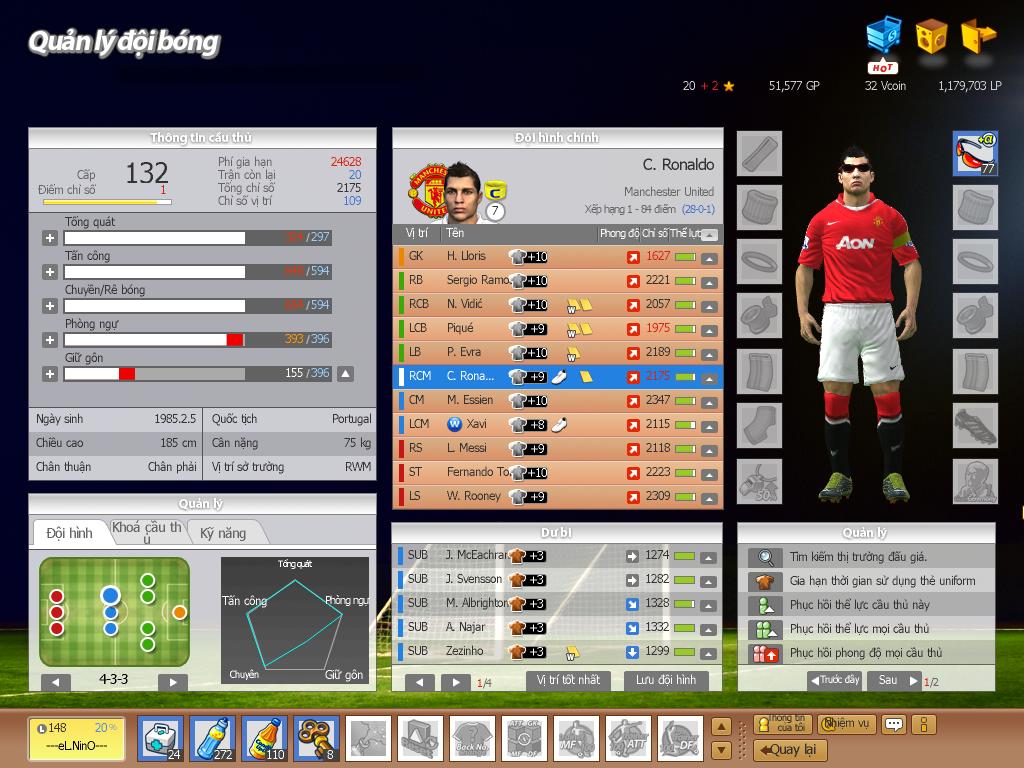The image showcases a still from a video game screen. In the upper right corner, a character dressed in white shorts, a red short-sleeved shirt, and black, red, and white socks is visible. The screen's text appears to be in a foreign language, with the upper left corner displaying "Kwan Lee Doi Bong." The game's context reveals that the player, C. Ronaldo from Manchester United, is featured prominently. Several scores or statistics, such as "1627222120571975," are listed to the left of the character. Additional text in the upper left corner reads "Thong Tin Kao Tu," likely indicating players' names or game-related information. Names like "Thong Kwat," "Thong Kong," "Cheyenne De Bong," and "Thong Myur Yi Gong" are visible, potentially representing other characters or players. At the bottom of the screen, a series of icons are displayed, including a first aid kit, a water bottle, another beverage, and a key, all of which are illuminated.